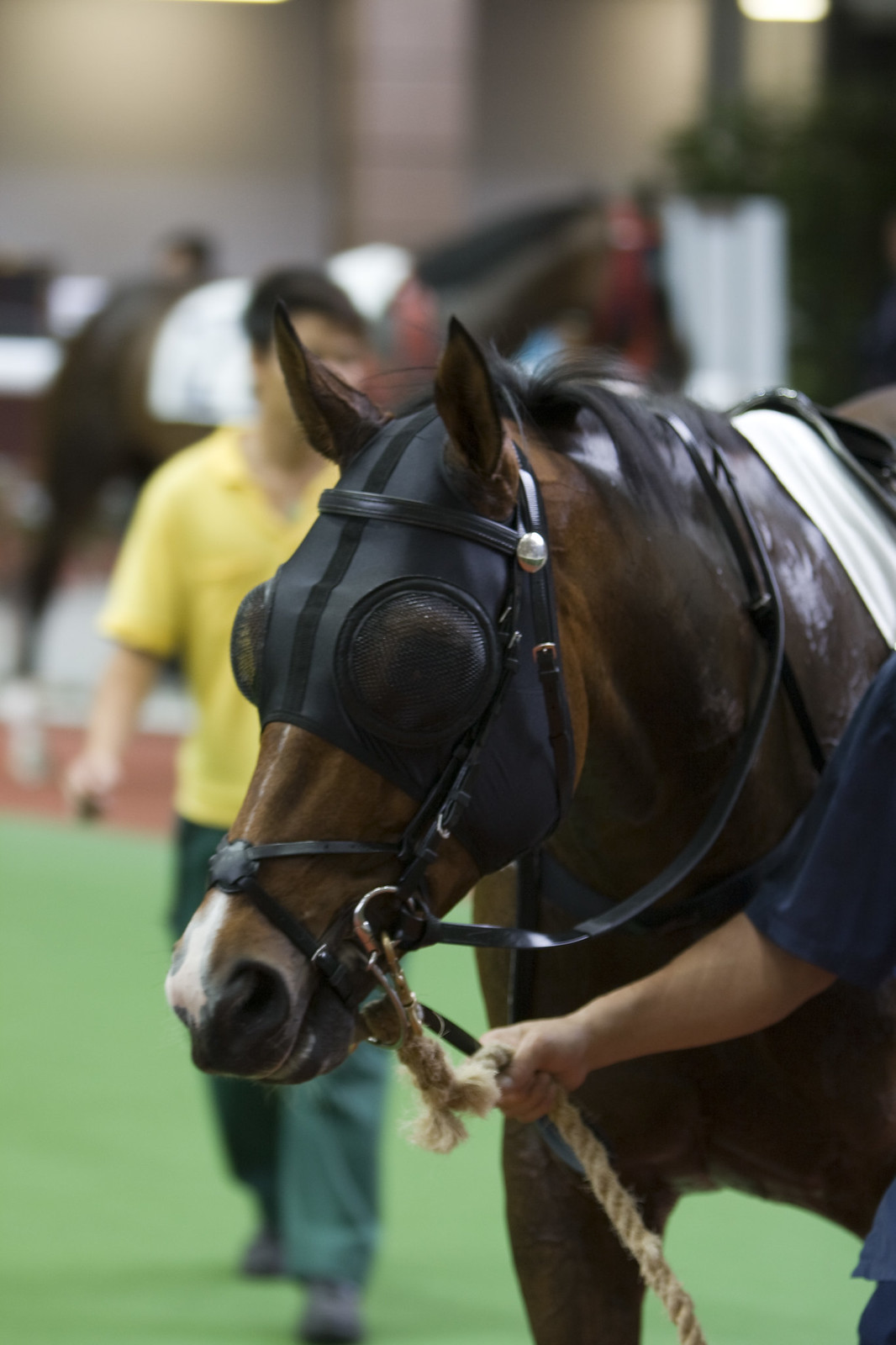In the image, we see a scene at a racing facility. A prominent feature in the foreground is a well-groomed, dark chocolate brown horse adorned in racing attire, including a saddle and a protective mask with mesh coverings over its eyes. The horse is held by a man wearing a blue shirt, visible by his arm gripping the reins. The background is blurred due to the depth of field, making the scene behind the horse less distinct. However, we can discern a man in a yellow shirt and green pants (or possibly jeans) walking towards the camera. Additionally, another horse is barely visible in the distance, distinguishable by a red accessory over its face and a riding blanket. The ground in the area appears to be a mix of a green surface and a brown walkway, adding to the atmosphere of this active racing venue.